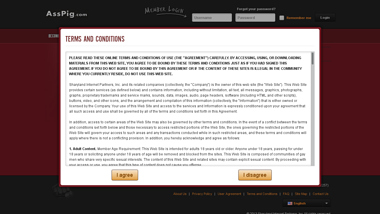In this image, we see a screenshot of a computer screen with a distinct layout and various elements. The background consists of a black border at the top and bottom, with dark red on the sides. Centered within this screen is a white rectangular box containing text.

At the top left corner of the white box, the text "Terms and Conditions" is prominently displayed in red. Below this header, the box is filled with several paragraphs of text written in black, detailing the terms and conditions.

At the very bottom of the white box, there are two small yellow rectangles serving as buttons. The left rectangle is labeled "I agree," while the right one says "I disagree," indicating the user's options for accepting or declining the terms and conditions. These buttons suggest a requirement for user interaction to proceed.

Above this white box, within the black border area at the top of the screen, the text "ASS pig" is displayed, presumably referring to a name or title relevant to the content. Also in the black bar area are two gray boxes, likely input fields for a username and password.

Overall, this screenshot captures a moment where a user is prompted to agree to terms and conditions, possibly as part of a login or setup process on their computer.